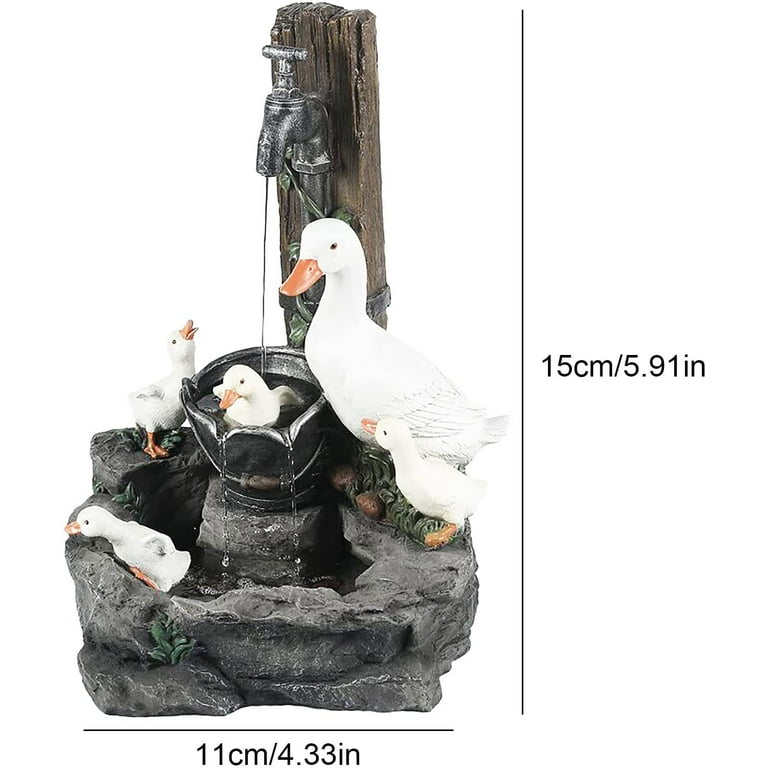The image showcases a detailed decorative piece resembling a miniature diorama featuring a group of white duck statues. Central to the scene is an improvised fountain setup with a stone bowl base, a wooden pole, and a faucet positioned on the pole, dispensing water into a metal bucket below. The fountain is populated with five animated ducklings and their attentive mother duck, characterized by their vibrant white feathers, orangish-yellow beaks, and matching feet. The ducklings are depicted in various adorable activities: one peering out, another reaching for food, and others seemingly enjoying the water, adding an element of liveliness to the piece. The diorama measures approximately 15 centimeters vertically and 11 centimeters horizontally.